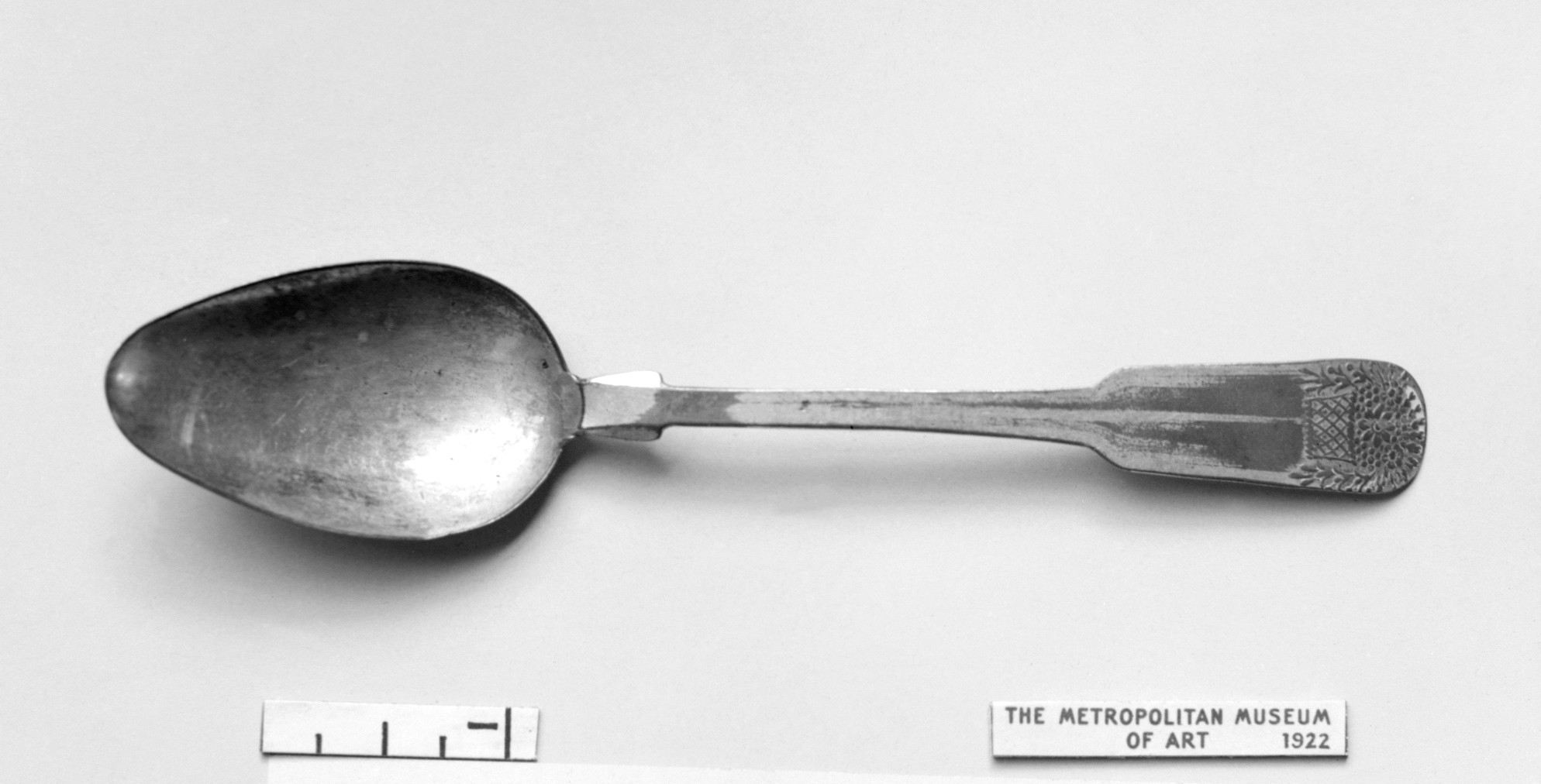In this full-color, horizontally rectangular photograph, we see a prominently displayed artifact from the Metropolitan Museum of Art. The background is off-white, emphasizing the monochrome theme of the image. Positioned near the center of the photo is an old, worn silver spoon with a large, round bowl and an extended handle featuring a small decorative detail at the tip. Positioned towards the bottom left, three letters, possibly "MCI," are faintly visible. In the bottom right corner, there's a rectangular plaque or pin reading in all caps: "THE METROPOLITAN MUSEUM OF ART, 1922." This image highlights the historical and possibly ancient nature of this spoon, suggesting its significance within the museum's collection.